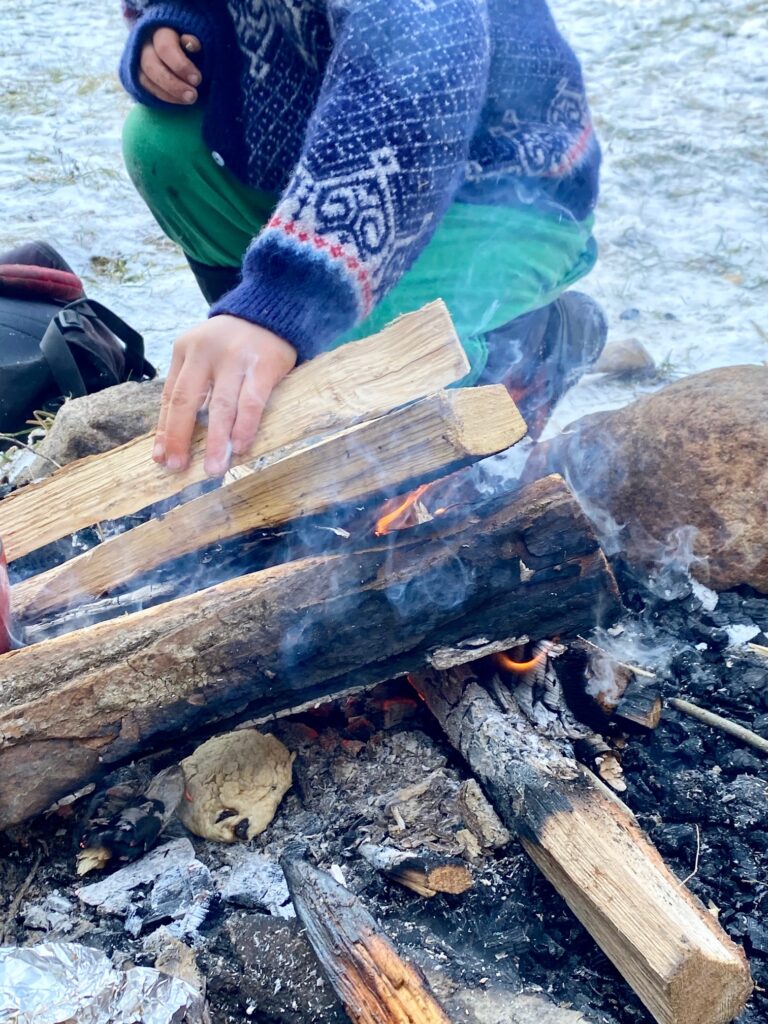A close-up photograph captures an outdoor campfire, showcasing intricately arranged split logs. The burning wood is piled methodically, with the lower logs already halfway reduced to a grayish ash. Vibrant orange flames dance upwards from the center, with tendrils of smoke curling off a blackened, charred log at the core. The upper logs, freshly split and yet to catch fire, await their turn to burn. A hand reaches into the frame, belonging to a person kneeling to place a new log onto the fire. Though only partially visible, the individual dons green pants and a blue patterned sweater adorned with white diamond shapes and red accents at the wrists. The fire pit is encircled by large tan boulders, creating a rustic boundary. In the background, the ground appears whitish, suggesting a light dusting of snow, with sparse green patches hinting at a cold, wintry setting.